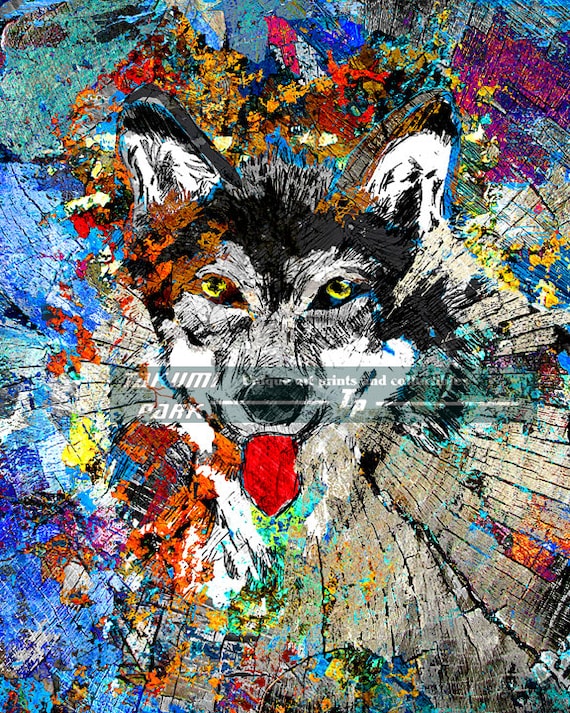This artwork is a vibrant, abstract painting depicting the face of a wolf, possibly resembling a husky or an Alaskan Malamute. The wolf, with its striking yellow eyes and red tongue protruding, is primarily black and white with distinct color splatters throughout the background. The fur around its eyes and nose is framed with white while the rest of its head and the tips of its ears are shrouded in black. The background is a chaotic explosion of colors, with blue, purple, and orange dominating the bottom left, teal and blue in the upper left, and magenta splatters in the upper right. The bottom right features a distinct gray texture. An ink mark crosses over part of the face, adding to the abstract nature of the piece. There is also a watermark that reads "Takumi Park, unique art prints in collectibles," with the letters "TP" flanked by lines, contributing a subtle touch of authenticity to this highly detailed and dynamic visual experience.